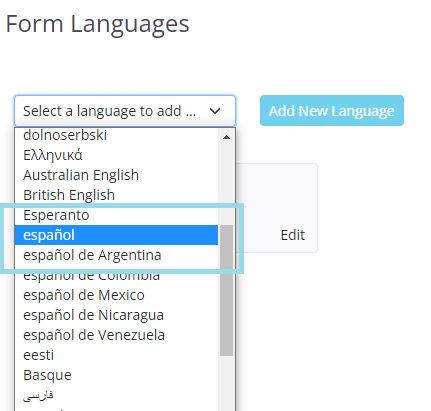The screenshot depicts a language selection interface on a website, presented against a white background. At the top left corner, the text "Form Languages" is displayed in a pale black font. Directly below this title, the instruction "Select the language to add" is provided. This interface appears to be part of a form creation tool, enabling users to choose their preferred language for filling out and interacting with the form, ensuring accessibility for a diverse audience.

The primary focus of the screenshot is a dropdown or scrolling list of various languages, arranged alphabetically. The list includes a wide range of languages and dialects. Some visible entries are "Don't don't know Serbiki Derbski," "Australian English," "British English," "Esperanto," and multiple variants of Spanish such as "Espanol," "Espanol de Argentina," "Espanol de Colombia," "Espanol de Mexico," "Espanol de Nicaragua," and "Espanol de Venezuela." A light blue rectangle highlights specific options in the list: "Esperanto," "Espanol," and "Espanol de Argentina," indicating that these languages might have been previously selected or are being recommended for selection. 

The design suggests the purpose is to facilitate the addition of multiple languages to ensure that form content is comprehensible to users from different linguistic backgrounds.